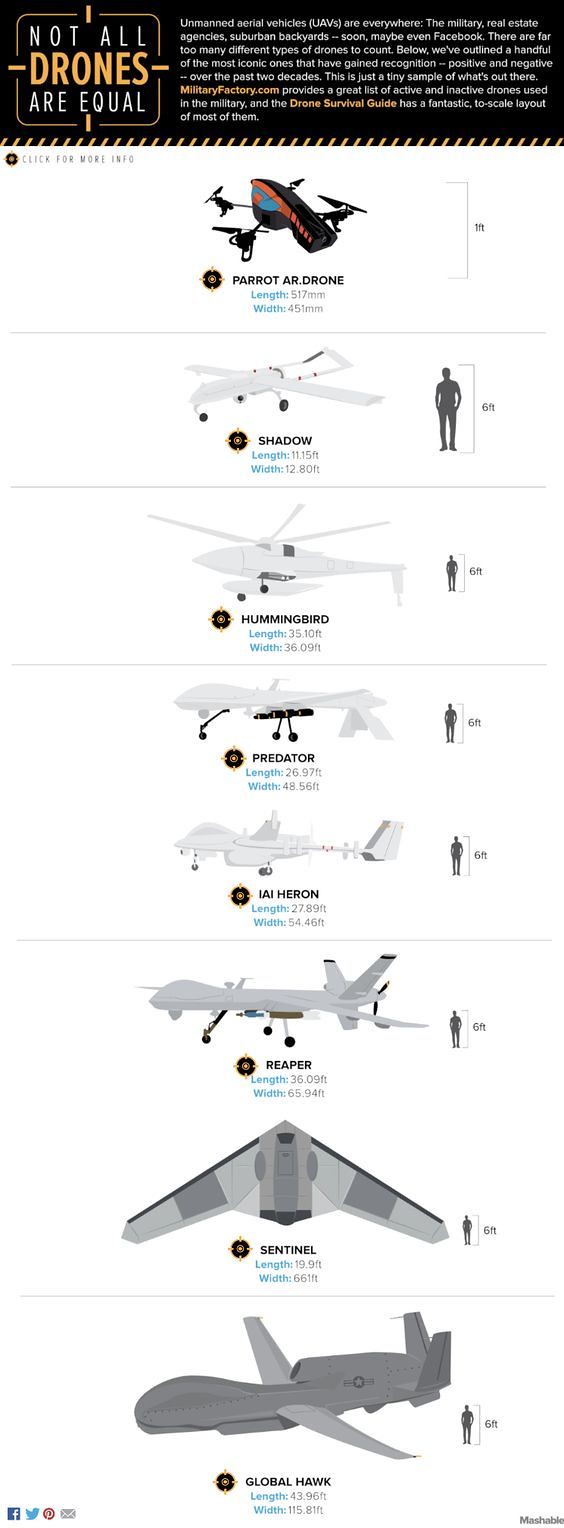The image is a vertically oriented diagram or illustration from an instructional manual or textbook, primarily using a black and white color scheme. At the top, there's a black banner with a yellow-trimmed square on the left side, containing the text "Not all drones are equal" written in gold and white. Below this, a white-on-black text block provides information about unmanned aerial vehicles, explaining their prevalence and various specifications.

The diagram organizes the drones into eight distinct panels, each depicting different types of drones, from the smallest to the largest. Each drone is illustrated alongside a six-foot-tall human figure for size comparison. The drones include:

1. **Parrot AR Drone** - Approximately one foot tall.
2. **Shadow Drone** - Resembling a small plane, about six feet long.
3. **Hummingbird Drone** - Details are less clear here.
4. **Predator Drone** - Followed by a short descriptive text.
5. **Heron Drone** - Accompanied by some text that’s hard to read.
6. **Reaper Drone** - with brief descriptive text.
7. **Sentinel Drone** - Also with some accompanying text.
8. **Global Hawk Drone** - The largest, measuring 44 feet long and 116 feet wide.

This detailed diagram serves as a comparative guide to understanding the different sizes and types of drones, emphasizing that not all drones are equal.